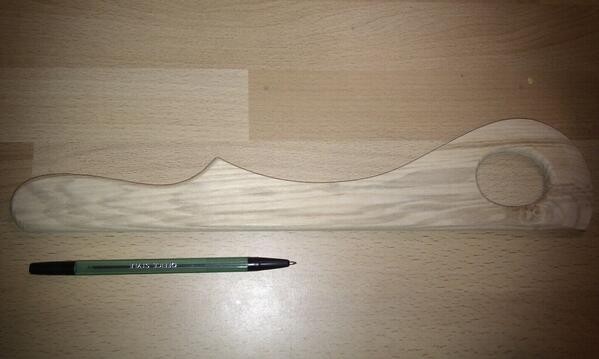The image features a light-colored wooden tool or utensil, possibly used in furniture making or as a stirring implement. The object exhibits a distinct design with a central handle that has a pointed middle, resembling a club, but with a flattened top. The top section includes a hole, potentially for functional use. The handle features grooved markings towards the bottom, making it ergonomic for holding.

The wooden material displays visible grain patterns, indicative of tree age markings, showcasing the natural beauty of the wood. The utensil appears clean and well-maintained, placed on a floor with a similar tan wood or linoleum finish, creating a harmonious visual effect. Positioned beside the object is a black pen, approximately half its length, likely included to provide a size reference for the viewer.